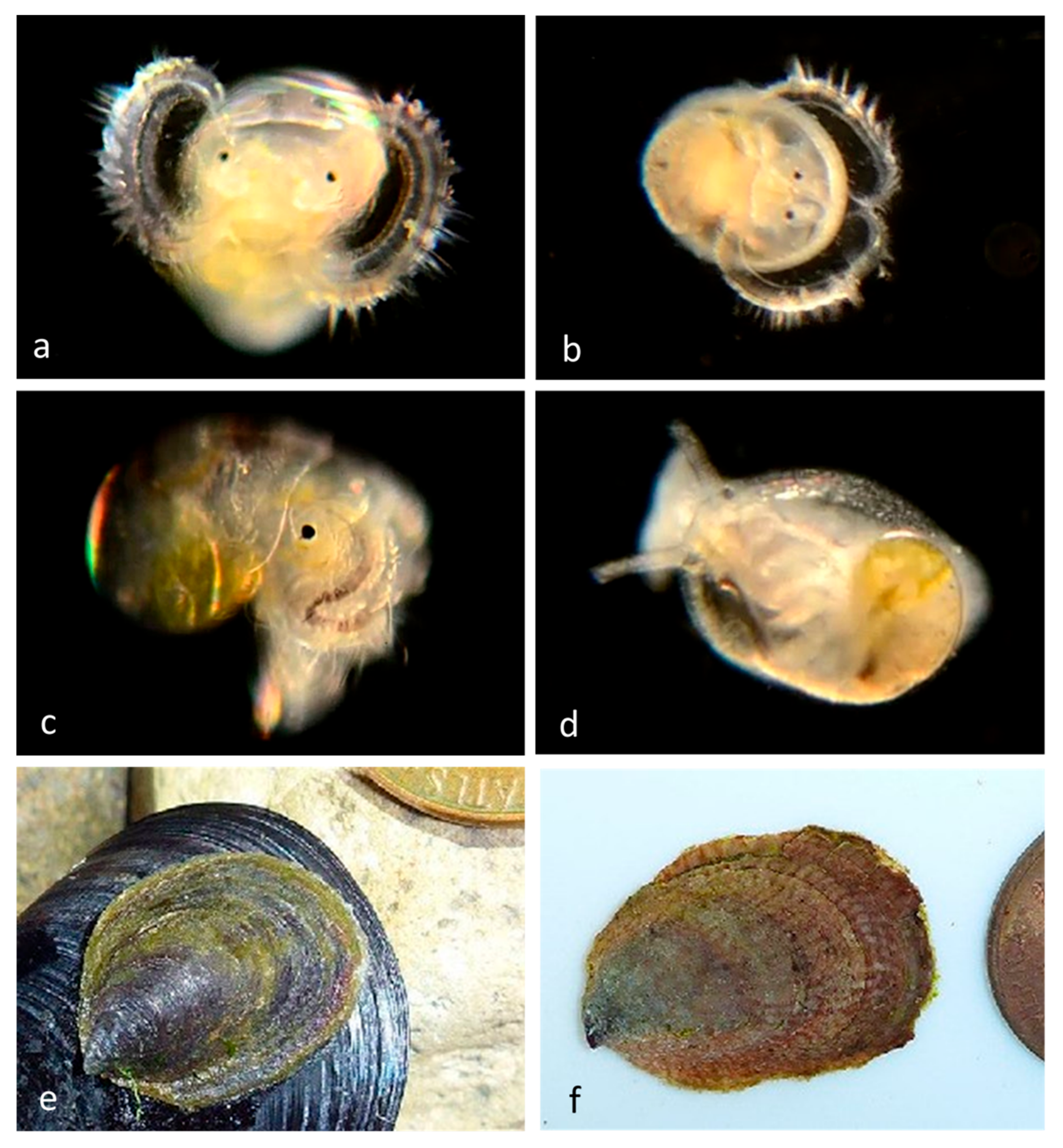The image is composed of six labeled photographs, A to F, arranged in two columns of three rows, showcasing the progressive development of what appears to be baby sea creatures, possibly octopi. 

In photograph A, the subject resembles a small, transparent sea creature with a jelly-like substance, displaying two distinct, beady eyes and yellow interior features. Moving to photograph B, the creature has grown slightly larger, maintaining its translucent appearance and yellow internal markings, resembling an egg yolk with tentacle-like extensions. For photograph C, the creature progresses further, showing more defined eyes and remaining jelly-like with visible yellow parts, hinting at its ongoing development.

Photograph D mirrors the prior stages but lacks visible eyes, continuing the theme of a transparent, yellow-highlighted marine being. In photographs E and F, the focus shifts to shells; E depicts a blue and green shell, while F features a brownish shell, suggesting either different developmental stages or different types of sea creatures. This series likely chronicles the development of these marine animals, transitioning from their early life stages as pods to their eventual encasement in shells.